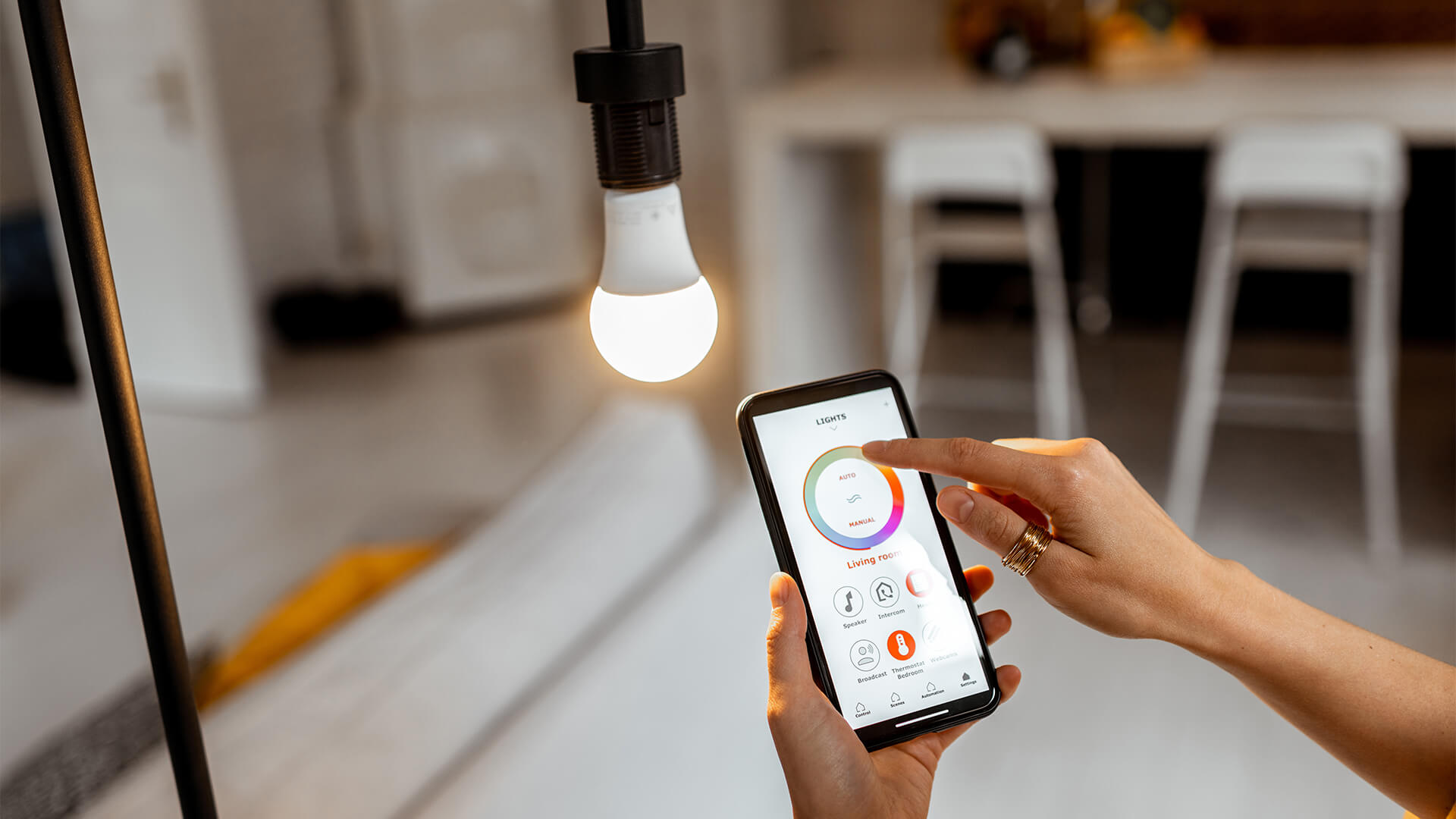The photograph depicts a person adjusting the luminosity of a smart light bulb using a smartphone in what appears to be a kitchen setting. The central focus is a luminous light bulb, hanging down from a black metal lamp cord, just above the phone. The phone screen displays a rainbow-colored circle being toggled by the person's index finger, likely to control the light's color and brightness. The phone interface also shows several icons at the bottom, including a music note, a house, a human figure, and a thermometer, with the latter being highlighted in red.

In the blurry background, a white wooden table with two tall, white backed stools is visible, as well as an assorted item atop the table. To the left, there's an open door with a gold handle and a yellow object on the floor. Additionally, a black pole is discernible on the left side of the image. The person adjusting the light has a gold ring on their thumb, further emphasizing the interaction between the smartphone and the intelligent lighting system.